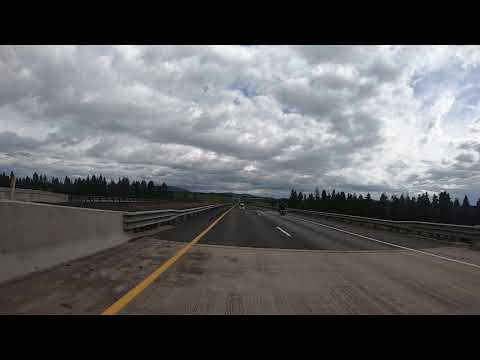The photograph captures an empty, paved highway with two clearly defined lanes. On the left, a solid yellow line and a metal barrier demarcate the road's edge, while a dashed white line runs down the middle. The bottom of the image shows significant dirt and gravel, suggesting the road may need repairs. The sky overhead is densely overcast, with the sun barely peeking through the clouds in the upper right. In the distance, several vehicles can be faintly seen, including one white car on the left and a darker vehicle on the right. Farther away, coniferous trees with pointed tops outline the horizon, and there are mountains to the left side of the image. Despite the overcast weather, no precipitation is evident, and the scene suggests a rural setting, potentially with a bridge or other light concrete structure present in the background.